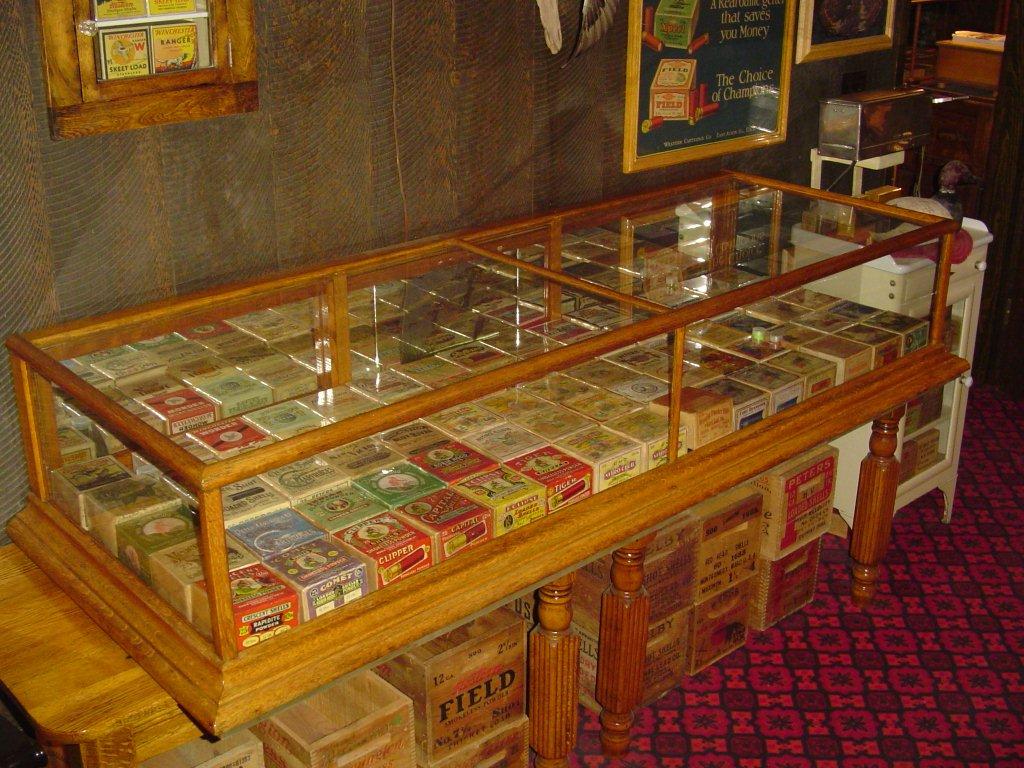The image depicts a glass cabinet with a wooden frame, resting against a dark wooden plank wall. Inside the cabinet, neatly displayed boxes of ammunition, including shotgun shells, are organized meticulously. Below the glass case, there are larger boxes holding additional ammunition. The cabinet is set on a reddish-purple, velvet-like carpet that evokes a vintage 1970s aesthetic. To the right of the case, a short white shelf supports a silver machine. The wall behind features a large, wood-framed vintage poster advertising shotgun shells and a smaller gold-framed piece. On the far left, another wooden frame showcases small photographs depicting the tops of the ammunition boxes.